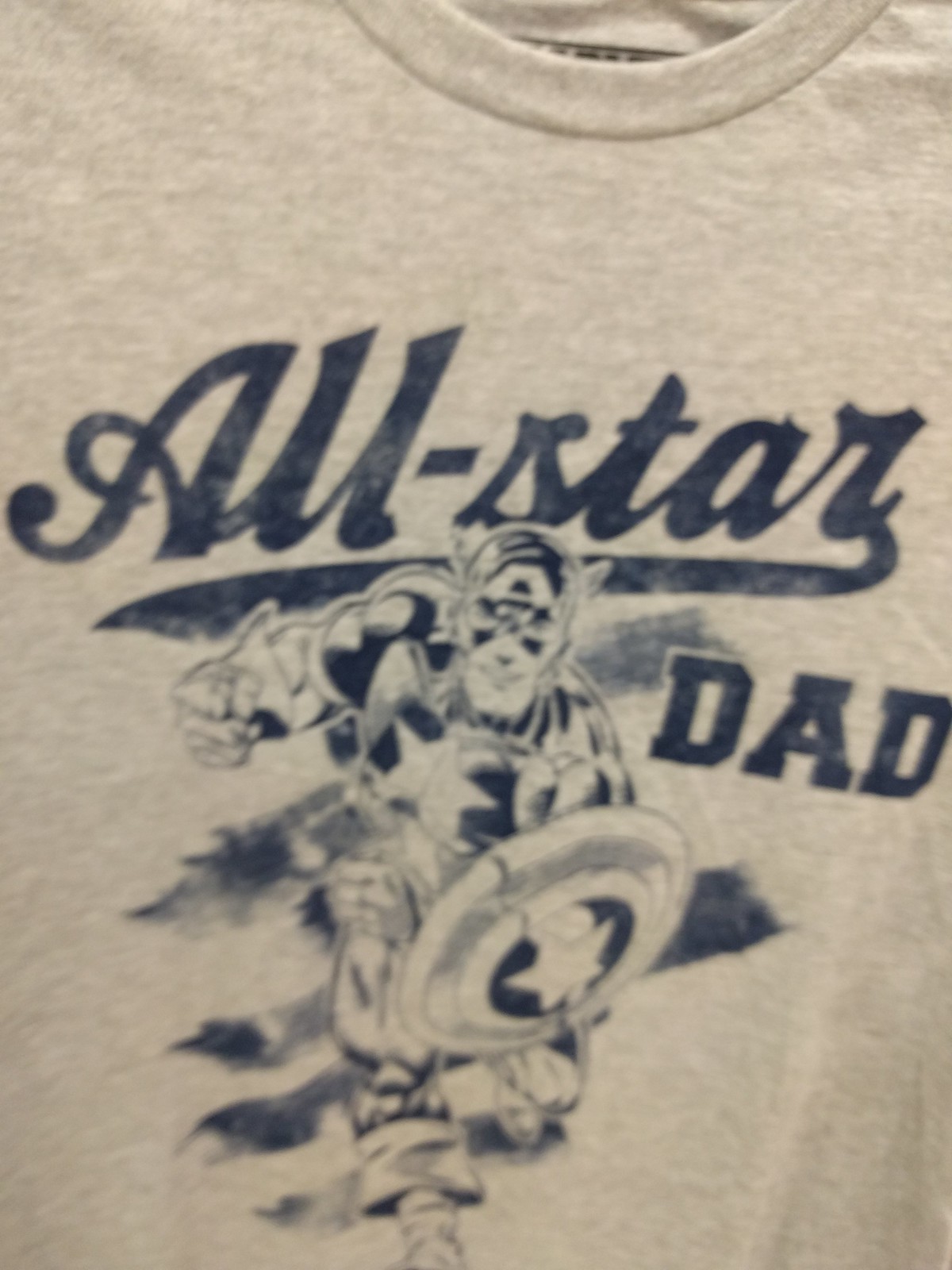This is a close-up photograph of an off-white t-shirt with a detailed graphic in dark navy blue ink. The t-shirt features the text "All-Star Dad" in a cursive, sports jersey-type font, where "All-Star" is hyphenated, and "Dad" is in all caps. Centered below the text is a dynamic illustration of a character resembling Captain America, depicted in a mix of white and dark blue with white accents. The character is portrayed in a forward motion, seemingly walking or running toward the viewer. He wears a costume similar to Captain America's, with a star emblem on the chest, a leotard combined with baggy pants that highlight his bulging leg muscles, and a mask with a capital 'A' and blue accents. His shield is prominently displayed with a white star and circular blue accents. Blue splotches and a flame effect behind the character enhance the sense of motion. This detailed and vigorous design captures a superhero-themed tribute to dads.